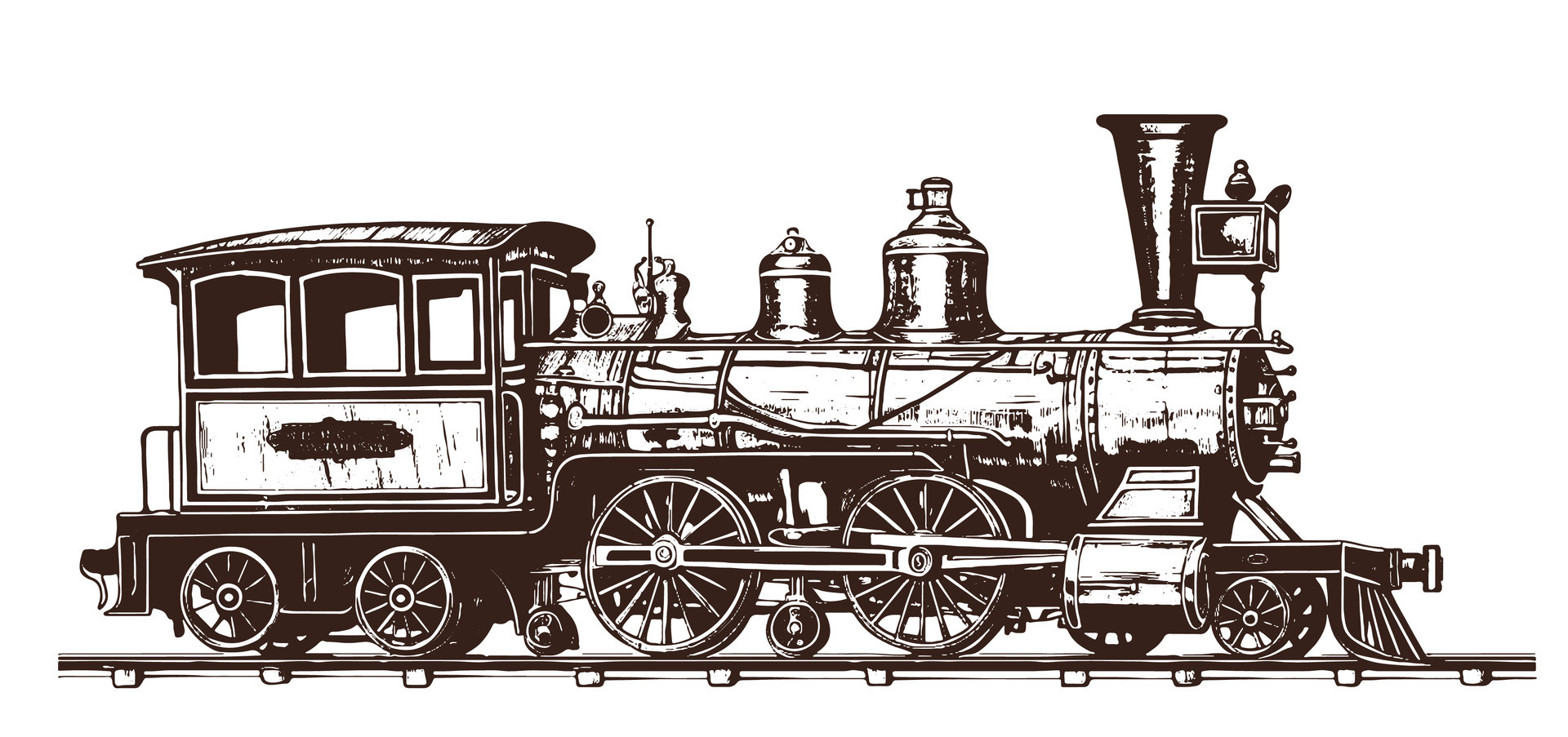This detailed black-and-white illustration depicts a stationary train on a single set of tracks against a plain white background. The front of the train, which is the primary focus, showcases a highly detailed and larger-than-average conductor's booth. This booth is equipped with three bells and a steam outlet. The train has a total of three sets of wheels: two larger sets in the middle, one smaller set at the front, and two medium sets at the back, supporting an adjoining cart. The cart features three windows and a metal plaque on its side, possibly engraved with the train's name, though the text is too small to decipher. Overall, this intricate hand-drawn image captures the essence of a traditional train with impressive clarity and detail.